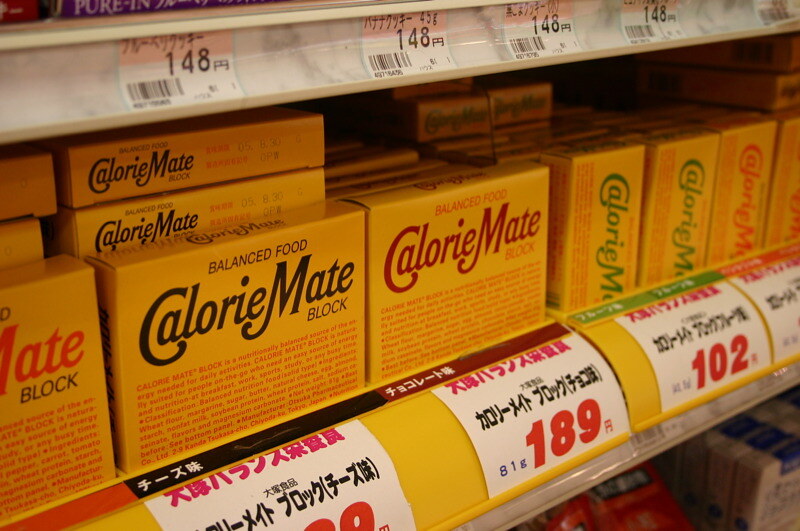The image depicts a light beige, ridged, metal grocery store shelf, lined with uniform yellow brick-shaped boxes of "Calorie Mate Block" products. The boxes feature the text "balanced food" in smaller font, while the larger text "Calorie Mate" appears prominently. The text color on the boxes varies, including red, green, orange, and black. Beneath the product labels, large red text details additional information. The shelves display white tags with barcodes and numbers, suggesting pricing details in a foreign language. Some tags show prices like 189 and 102, possibly indicating different prices for the varying box colors. Larger sale tags in red numbers are added to the shelf, indicating special pricing or promotions.